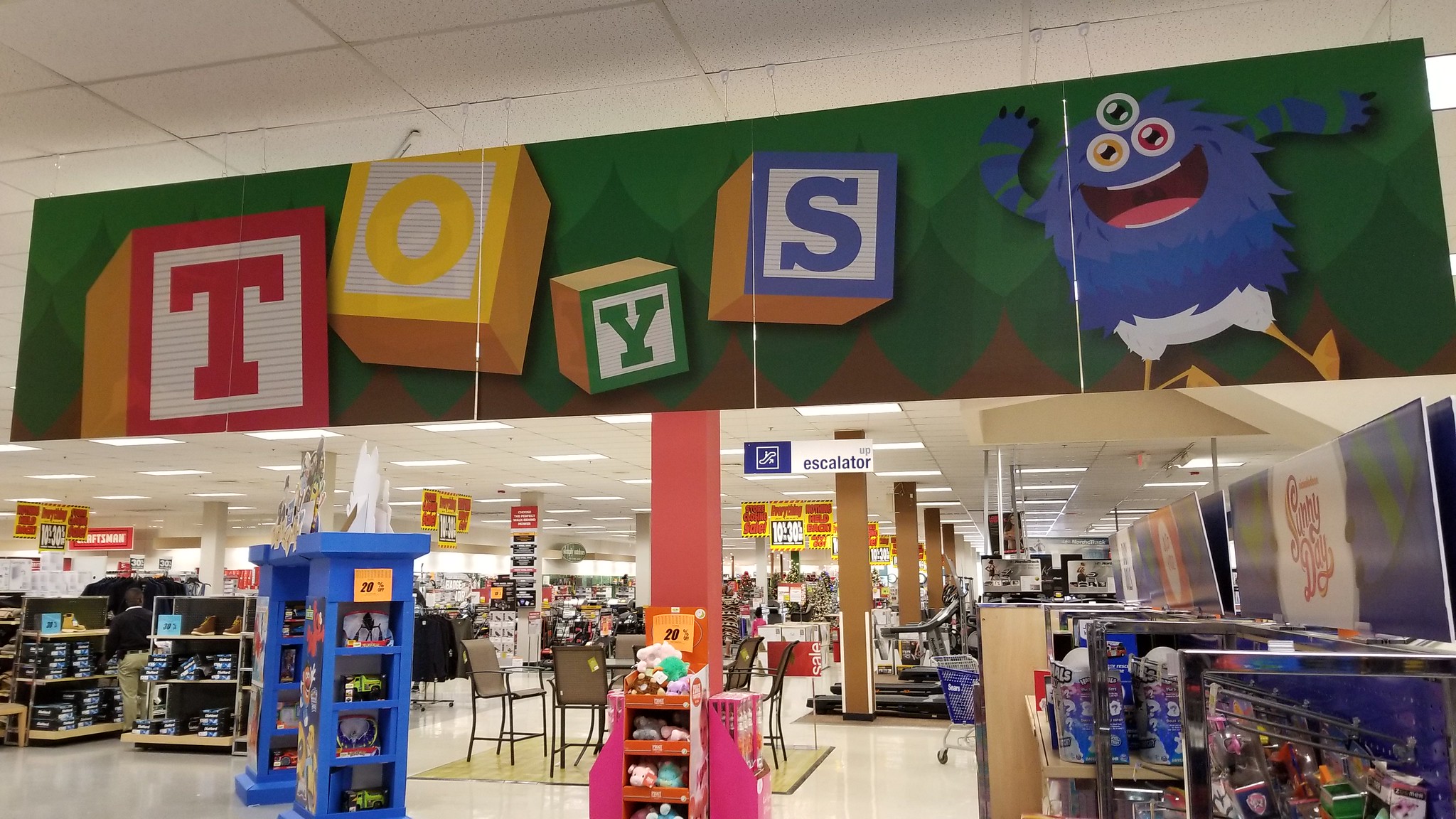The image depicts a vibrant toy store, likely situated in a mall, characterized by an open storefront. Prominently displayed at the top, suspended by white chains from the ceiling's white panels, is a large green sign that reads "TOYS," with each letter formed from colorful children's building blocks: a red T, a yellow O, a green Y, and a blue S. Accompanying the sign to its right is a cheerful, blue fluffy monster character. This whimsical creature has three eyes—each uniquely colored green, yellow, and blue—adorned with white pants or feathers and yellow duck-like legs. Below the sign, the bustling store features shelves brimming with toys and racks of clothing, particularly on the left side. There's an array of items, including discount signs and a table set for sale, amidst the neatly arranged aisles, under a spacious white-tiled floor.